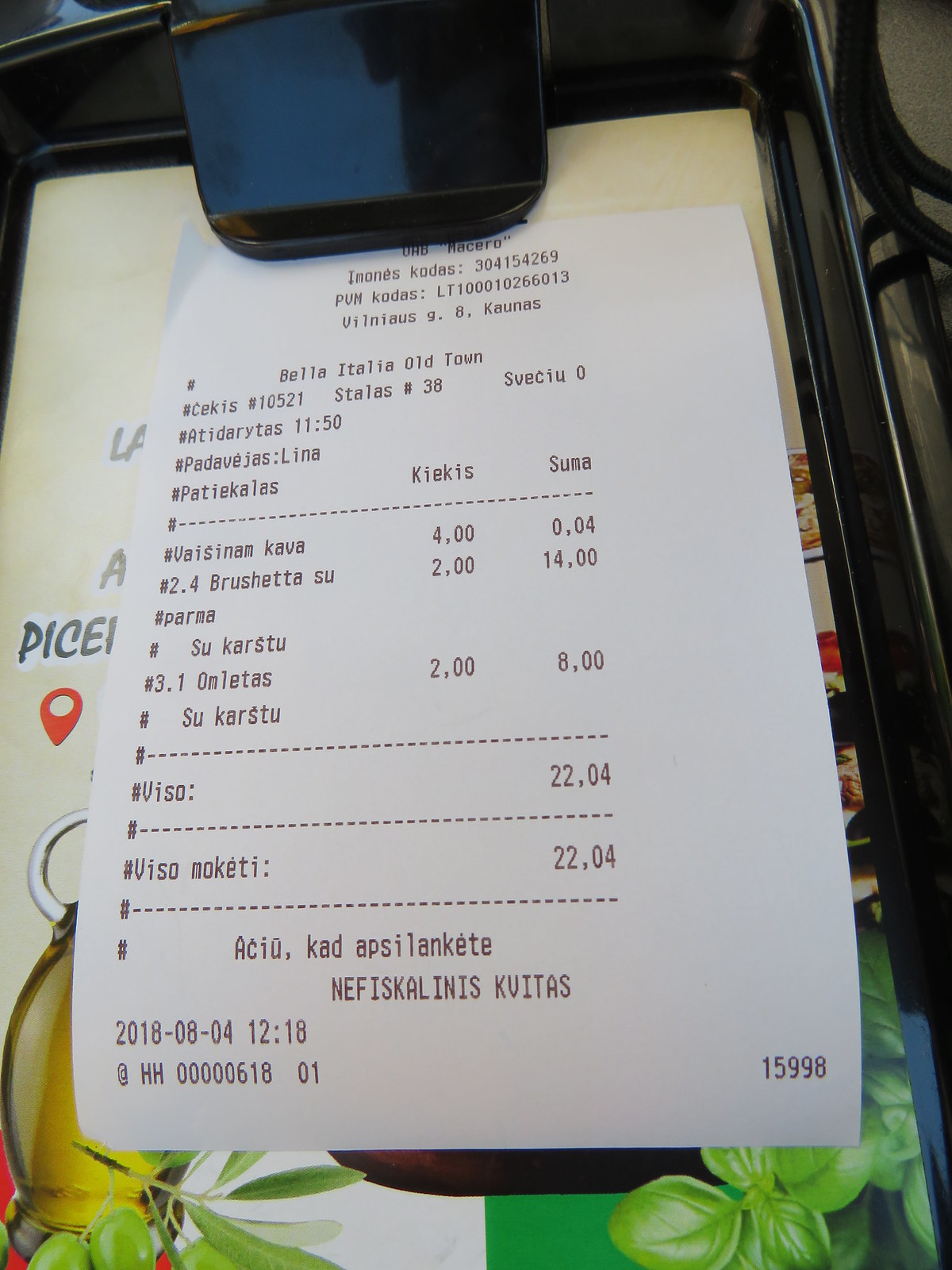The image displays a white receipt adorned with black writing, mostly in a language that appears to be Italian, given the visible text "Bella Italia Old Town". The receipt details several items including "bruschetta" and lists various prices, such as one item priced at 42 (currency unspecified). The receipt features dashed lines segmenting different sections and is dated "2018-08-04" with a timestamp of "12:18".

In the background, a menu is partially visible along with what seems to be a bottle of olive oil, surrounded by green olives and leaves, adding a touch of greenery to the scene. The entire setup rests on a black plate, with a matching black holder securing the receipt and menu in place. The overall backdrop has a manila-colored tone, complementing the sophisticated yet casual dining ambiance.